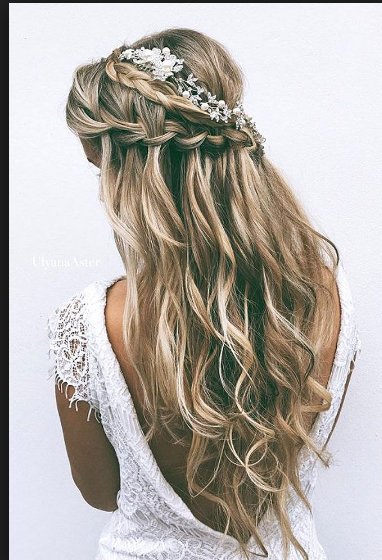This poster-sized, close-up photograph captures the back of a bride with long, wavy brown hair adorned with blonde highlights. Her hair cascades down her back, elegantly curling towards the bottom. Two loose braids frame the crown of her head, interwoven with delicate white baby's breath flowers, adding a natural, whimsical touch. She wears an open-back, white wedding gown with intricate embroidery and lace cap sleeves. The sheer, frayed fabric over her shoulders extends downwards, partly obscuring her exposed lower back. Her complexion is olive-toned, and she turns slightly to her left, her left eye barely visible. The stark white background emphasizes her intricate hairstyle and elegant dress, while the photograph itself is set against a contrasting black backdrop, highlighting the delicate details of this bridal portrait.